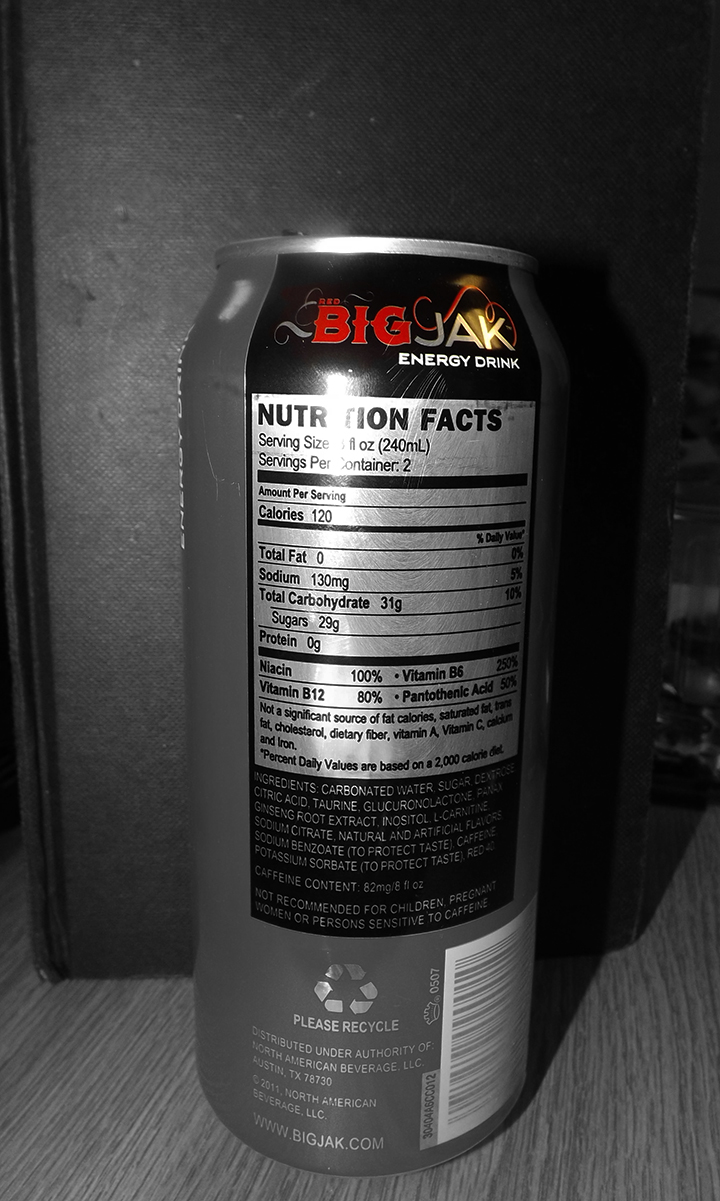The image depicts a can of Big Jack energy drink, specifically the back view displaying detailed nutritional information. The can is relatively tall, estimated at 16 ounces, and the photo is in black and white except for the can’s logo at the top, which is red. The label features nutritional facts indicating two servings per container, each serving being 120 calories. Key ingredients include carbonated water, sugar, dextrose, citric acid, taurine, glucuronolactone, and ginseng root extract. It also highlights an 82 mg caffeine content per 8 fluid ounces, totaling a substantial amount in the full can. 

The background of the image portrays a wooden table with apparent wood grain, and another object resembling a black checkbook. The nutritional label is silver on a black background, stating 0 grams of fat, 130 milligrams of sodium, 31 grams of total carbohydrates, 29 grams of sugar, and essential vitamins such as niacin, vitamin B12, B6, and pantothenic acid. The brand logo features ‘Big’ in an old-fashioned thick red font, while ‘Jack’ or ‘JAK’ is in a modern thin silver font. Additional details on the can include a recycling symbol at the bottom, the instruction to "please recycle," and a website link accompanied by a barcode.